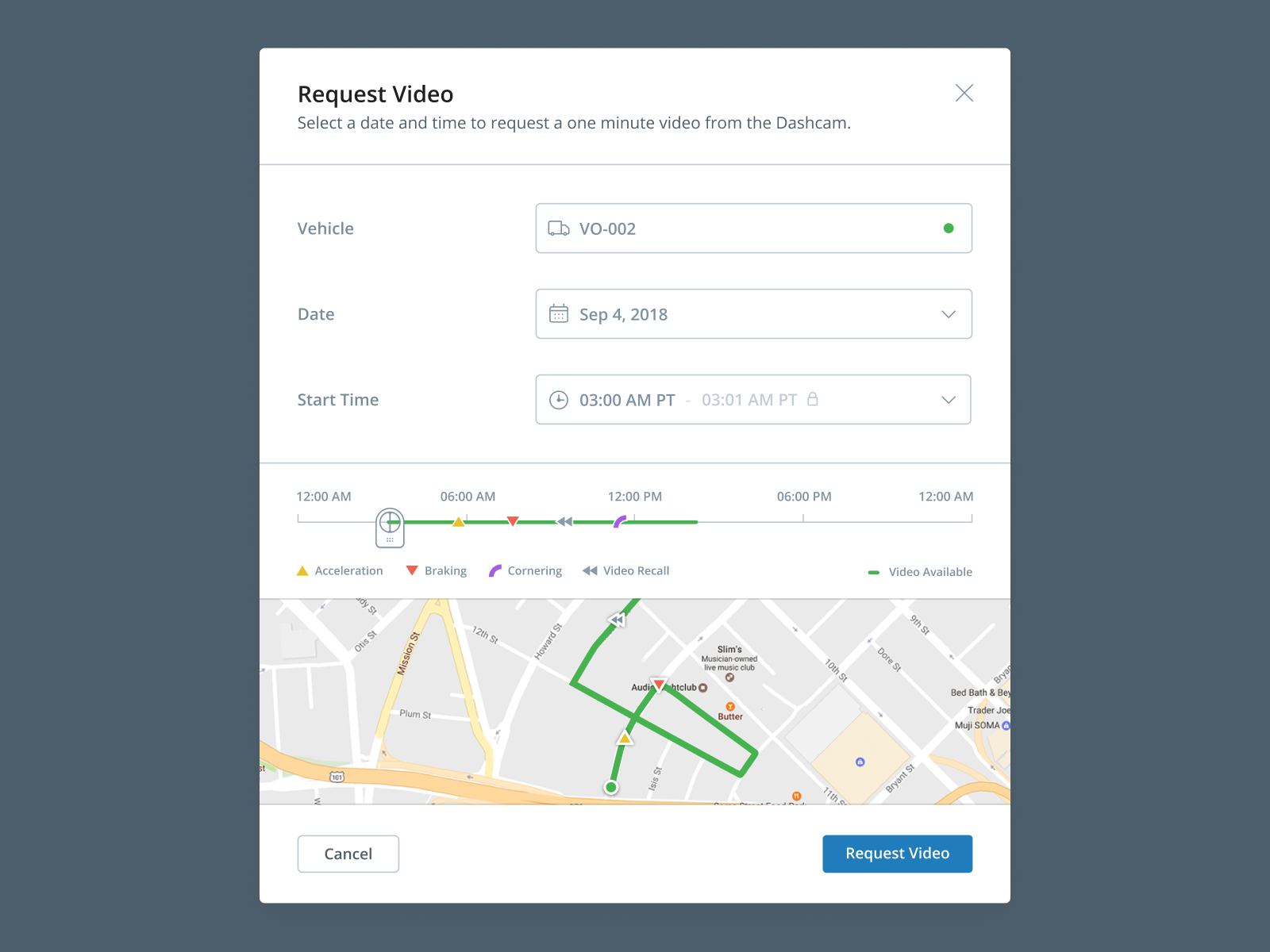**Caption:**

The screenshot features an olive green background with a prominent white box centered on top. At the top-left corner of the white box, "Request Video" is written in bold black letters. Opposite this, on the top-right corner, there's a gray 'X' icon meant for closing the box. Below the "Request Video" title, a gray text instructs, "Select a date and time to request a one-minute video from the dash cam." A thin gray line divides this instruction from the subsequent content.

Further down, on the left side, the word "Vehicle" is shown in gray text, accompanied by a rectangular gray box featuring an icon of a truck or car and the identifier "VO-002." To the right of this vehicle identifier, there is a small green circle. Below the vehicle section, the label "Date" appears in gray letters, followed by another gray box housing a calendar icon and the date "SEP 4, 2018." This section also includes a downward arrow for date selection adjustments.

Lastly, at the bottom of the white box, the label "Start Time" is displayed in gray, next to a gray box with a clock icon, set to "3 a.m. PT."